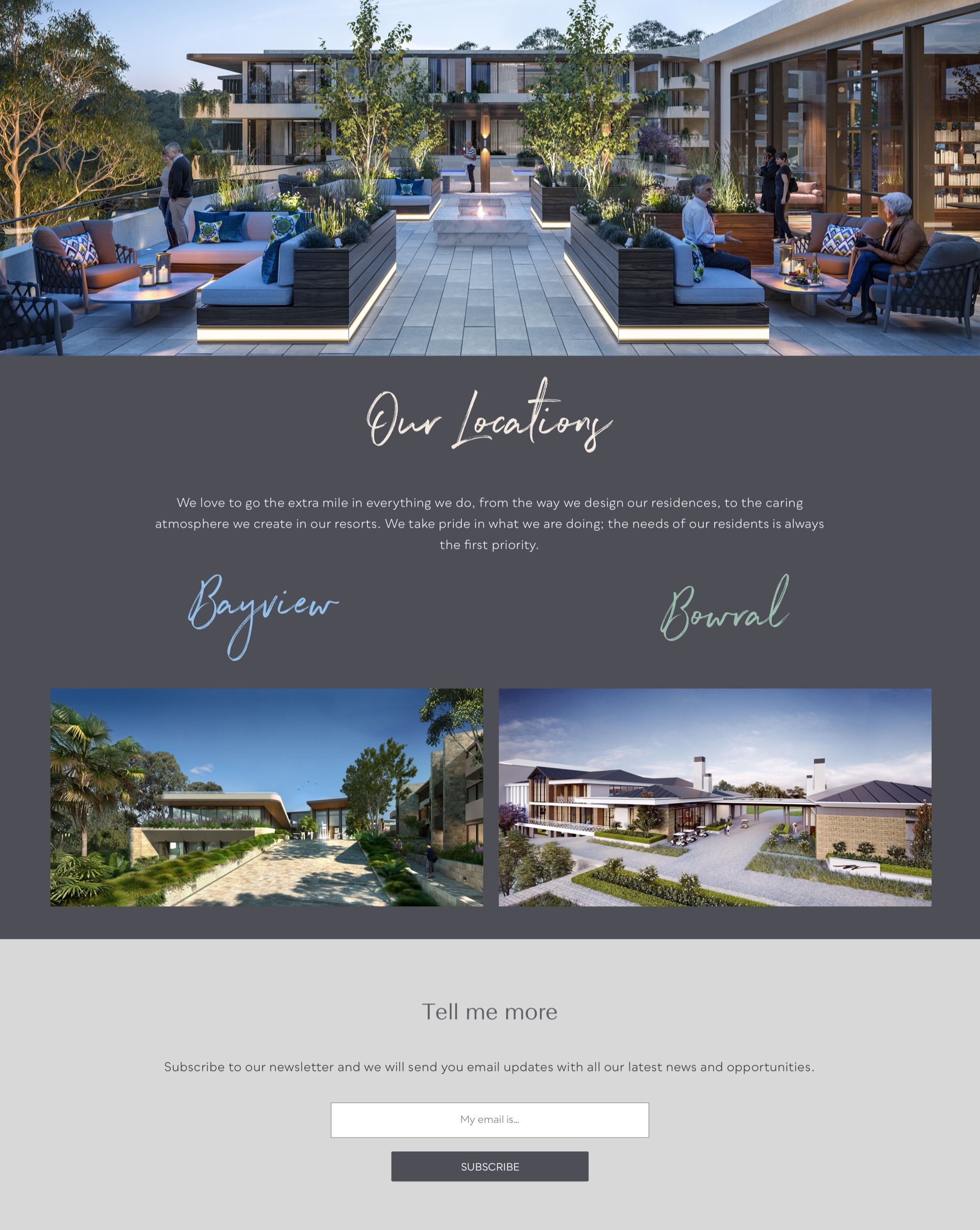This image is a snapshot taken from a real estate website. At the top of the image, there's a wide banner showcasing a series of luxurious homes, characterized by their substantial size and large windows. Below this banner, the website highlights its mission statement, emphasizing their dedication to going the extra mile in everything they do—from designing residences to creating a caring atmosphere at their resorts. They assert that the needs of their residents are always their top priority.

In the center of the image, there's a detailed description of their locations and services, radiating pride in their work. Toward the lower section of the snapshot, two additional pictures display various houses and buildings, further emphasizing the upscale and welcoming nature of their properties. The outdoor areas are depicted with greenery, including vibrant trees and groups of people comfortably seated on outdoor couches, reinforcing the community and leisure-focused environment they strive to foster.